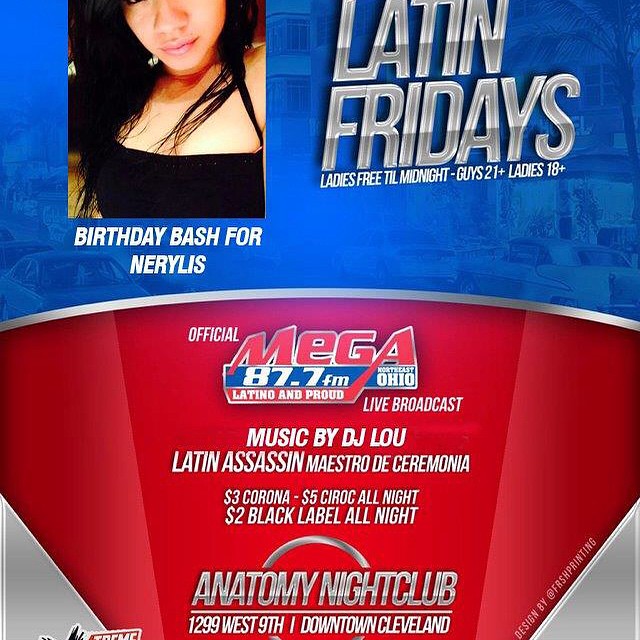The promotional poster for Anatomy Nightclub in downtown Cleveland features a vibrant design with blue, red, silver, and white elements. At the top, set against a blue background, bold silvery-gray text announces "Latin Fridays," highlighting that ladies get free entry until midnight, while entry requirements specify guys must be 21+ and ladies 18+. On the left side, a prominent selfie of a black-haired woman in a tank top advertises a "Birthday Bash for Neuralys." The bottom portion of the poster, primarily in red with white, blue, and silver fonts, promotes the "Official Mega 87.7 FM Latino and Proud Live Broadcast" from Northeast Ohio. The music lineup includes DJ Lou, Latin Assassin, and the Maestro de Ceremonia. Drink specials include $3 Coronas, $5 Ciroc, and $2 Black Label all night. The event takes place at Anatomy Nightclub, located at 1299 West 9th, downtown Cleveland. Additionally, a partially visible logo featuring a flying bird is positioned at the bottom left of the poster.